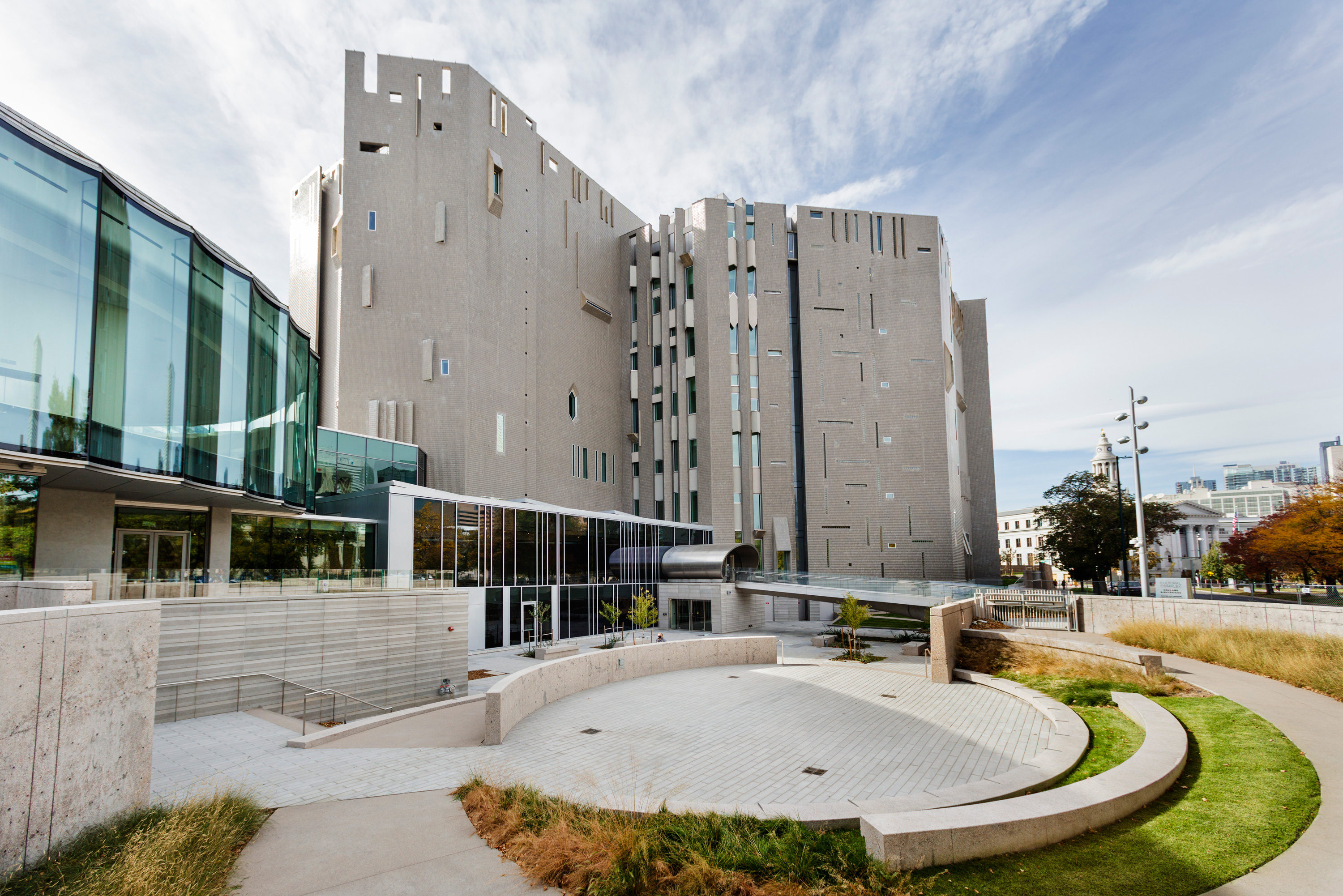This detailed image depicts the main courtyard area of what appears to be the Denver Art Museum. The centerpiece is a small, circular concrete amphitheater-like pad, surrounded by curved walkways and patches of green and brown grass. This round courtyard is encircled by multiple concrete barriers. Leading away from the courtyard are steps with railings that guide visitors towards a building entrance featuring glass doors.

To the left, the building showcases a second floor with nearly wall-to-wall, concave, large rectangular panes of glass arranged in a semi-circle. This structure is complemented by more glass and angular architecture. Further back, a footbridge with glass railings leads to an entrance that resembles a large metal tube.

To the right, the building is characterized by its unique angular design and assortment of differently shaped and sized windows, including rectangular and hexagonal forms. Beyond these structures, in the distance, the skyline reveals various gray apartment buildings, monument-like structures, and scattered power lines against a backdrop of blue sky peppered with white clouds.